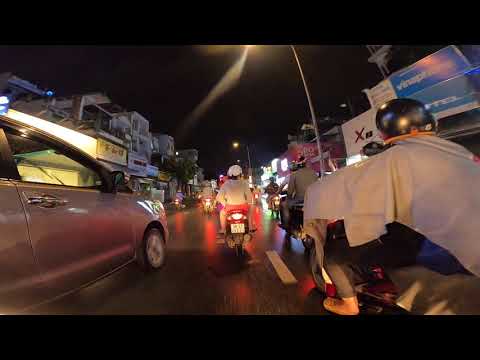This nighttime photograph captures a dimly lit street scene, marked by the intense blackness of the sky and the bright glare of a streetlight positioned centrally above. Directly in front of the camera, a moped or motorcycle with a red taillight is visible. To the immediate left, part of a silver sedan is seen, heading in the same direction. The wet pavement below reflects the lights of various vehicles, including several motorcycles scattered across the lane. Two of them are particularly noticeable on the right: one carries two riders, the rear one draped in a gray blanket and wearing a black helmet, while the other rider, closer to the camera, sports dark bottoms and a white shirt with a black helmet. The scene includes at least five motorcycles in total. Surrounding the street, there are buildings and shops on both sides, adorned with signage that potentially features Asian characters. The photograph's composition is framed by a black header and footer, emphasizing the nighttime gloom without borders on the sides.